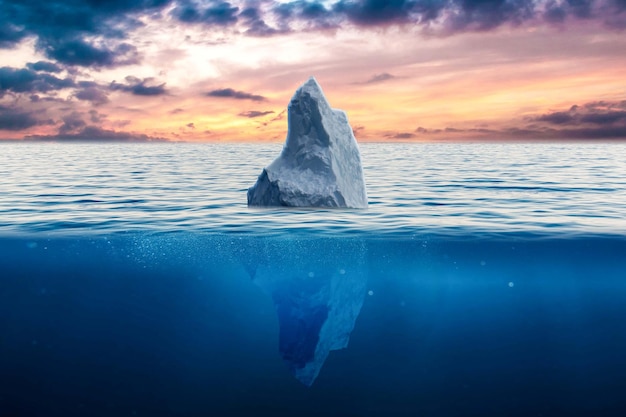The image, likely a painting due to its surreal elements, depicts a massive iceberg protruding from a clear blue ocean, occupying the central position of the composition. The jagged, uneven top of the iceberg rises above the water, while its submerged portion is visible beneath the surface, emphasizing its colossal size. The sky above is a blend of orange and blue hues, indicating either sunrise or sunset, with a dramatic touch of dark gray clouds creating a moody atmosphere. Toward the horizon, sandy hills with shades of brown and yellow can be seen. The water is so clear that air pocket bubbles are visible, but no marine life is present, adding to the ethereal and possibly science fiction-like quality of the image.